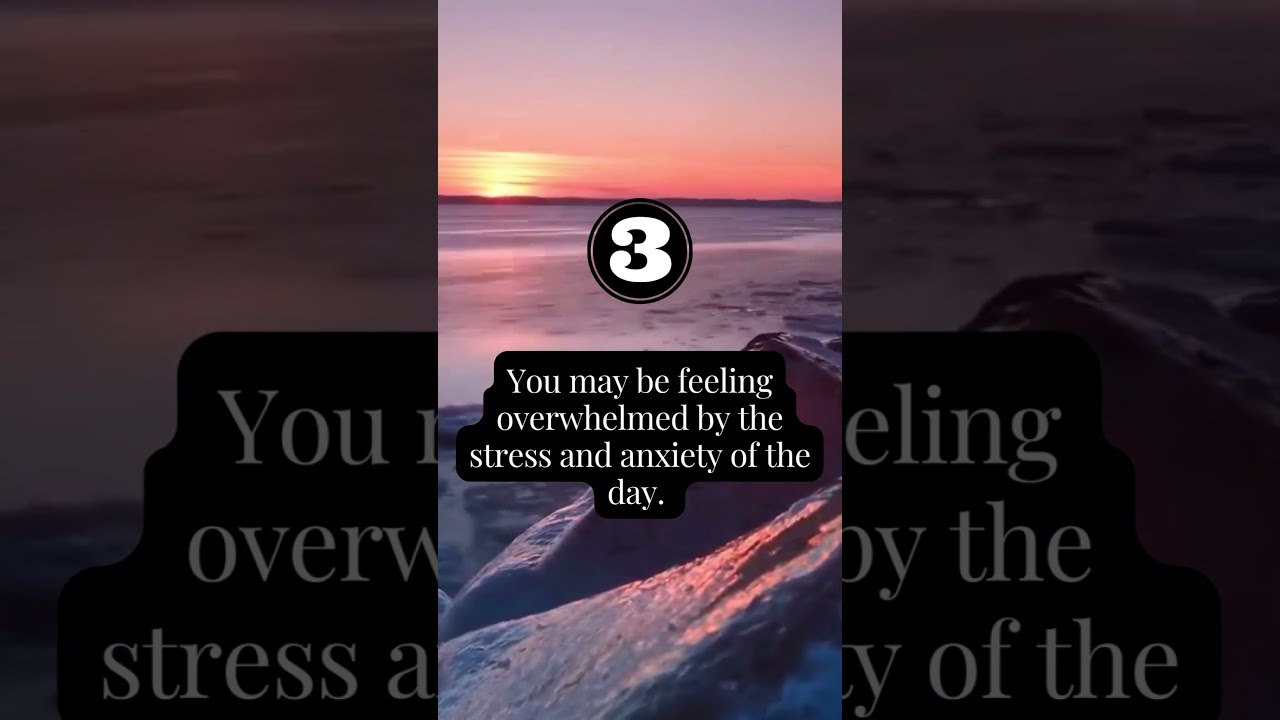The image is a meme structured in a triptych format, with the center panel displaying the focal point of the composition. The backdrop of the entire image is a color photograph taken at the ocean shore, featuring a rocky foreground leading to a sandy beach and then the water. The sky is painted in an orange hue, indicative of a sunset, with golden and pink tones illuminating the horizon. The central panel, which is in portrait orientation, prominently features a number three in white bold font within a black circular background. Below the number, in black text outlined in white and set against the same black background, the caption reads: "You may be feeling overwhelmed by the stress and anxiety of the day." The left and right panels of the triptych artfully magnify a portion of this text in a darkened tone, merging the photographic landscape with the superimposed message, thus creating an evocative scene that blends visual serenity with the contemplation of daily stress.